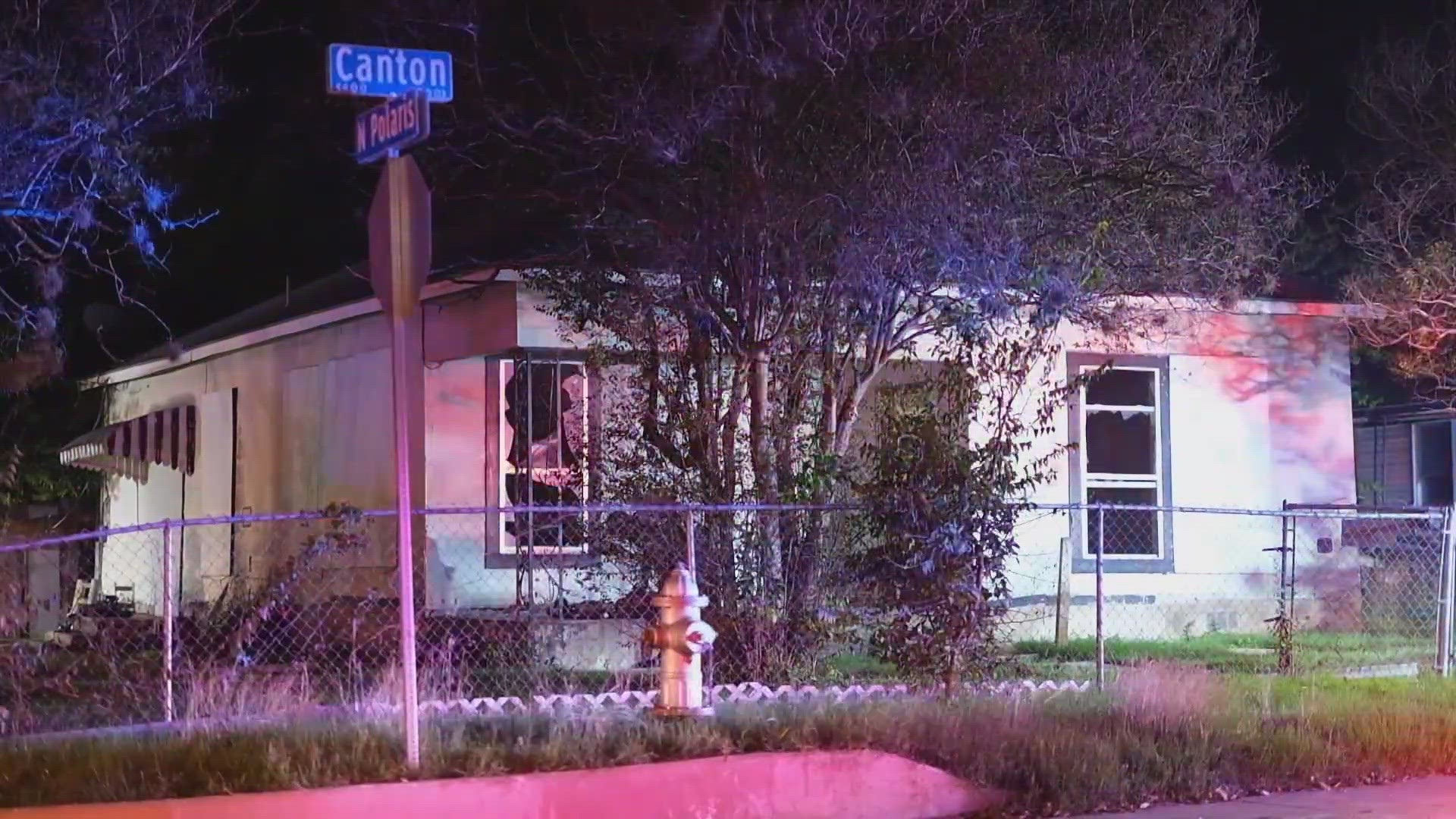This nighttime photograph captures the exterior of an older, single-story house, likely from the 1970s, with a flat roof and whitish cream-colored siding. The house features two windows flanking a central doorway, although a large tree in front partially obscures the view of the entrance. Additional trees stand around the property, and the house is enclosed by a metal chain-link fence approximately two to three feet tall. In front of the fence, a copper-colored fire hydrant is prominently visible toward the center of the image. A street sign, positioned to the left of the fire hydrant on a metal pole, intersects with a stop sign, displaying Canton and North Polaris as the cross streets on blue street signs. The house also has a red-and-white striped awning covering two chairs on the side. The scene is illuminated by streetlights, enhancing the visibility of details despite the nighttime setting. Grass along the sidewalk in front of the fence adds a touch of greenery to the urban landscape.